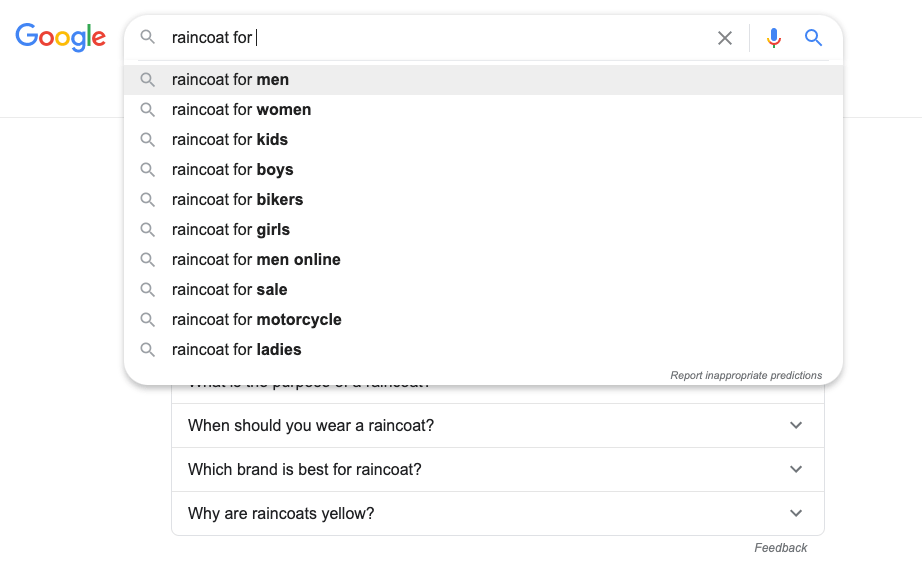This image captures the Google search homepage. In the upper left corner, the iconic multi-colored Google logo is prominently displayed. The main feature of the page is a search field where an individual is in the process of typing "Raincoat 4". This action has triggered a drop-down menu populated with search suggestions, listed as follows from top to bottom: "Raincoat for Men," "Raincoat for Women," "Raincoat for Kids," "Raincoats for Boys," "Raincoat for Bikers," "Raincoat for Girls," "Raincoat for Men Online," "Raincoat for Sale," "Raincoat for Motorcycles," and "Raincoat for Ladies." At the bottom of this menu, an option reads "Report Inappropriate Predictions."

Below the drop-down menu, there are four rectangles containing black text against a white background. The first rectangle is partially obscured by the drop-down menu. The subsequent entries read: "When should you wear a raincoat," "What brand is best for a raincoat," and "Why are raincoats yellow?"—the last of which poses an intriguing question.

In the lower right corner of the screen, there is gray text labeled "Feedback." The top right corner of the page features two blue icons: one representing a microphone and the other a magnifying glass, indicating tools for voice and text search, respectively.